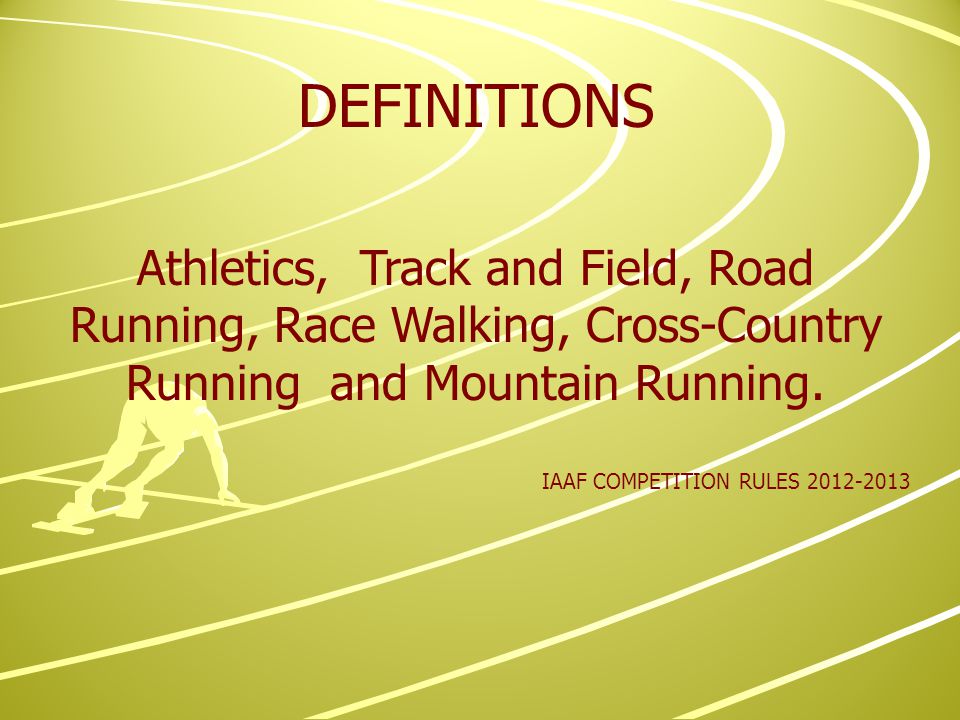The image depicts a PowerPoint slide featuring a detailed illustration of a circular running track. The background is predominantly yellow with varying shades, creating a dynamic representation of the track lanes defined by white lines, curving to form a pattern similar to a racetrack. Positioned at the top center of the slide, the title "DEFINITIONS" is prominently displayed in bold, dark red, all-capital letters. Below the title, the center of the image lists the following terms in a similar dark red font: ATHLETICS, TRACK AND FIELD, ROAD RUNNING, RACE WALKING, CROSS COUNTRY RUNNING, and MOUNTAIN RUNNING. Aligned slightly to the right, beneath these terms, is the smaller, still all-caps inscription, "IAAF COMPETITION RULES 2012-2013," maintaining the dark red color scheme. The green background features multiple curved lines, resembling a racetrack, with the tops of the curves facing right. Notably, an outline of a runner in light yellow is positioned in the lower left corner, adding to the athletic theme of the slide.